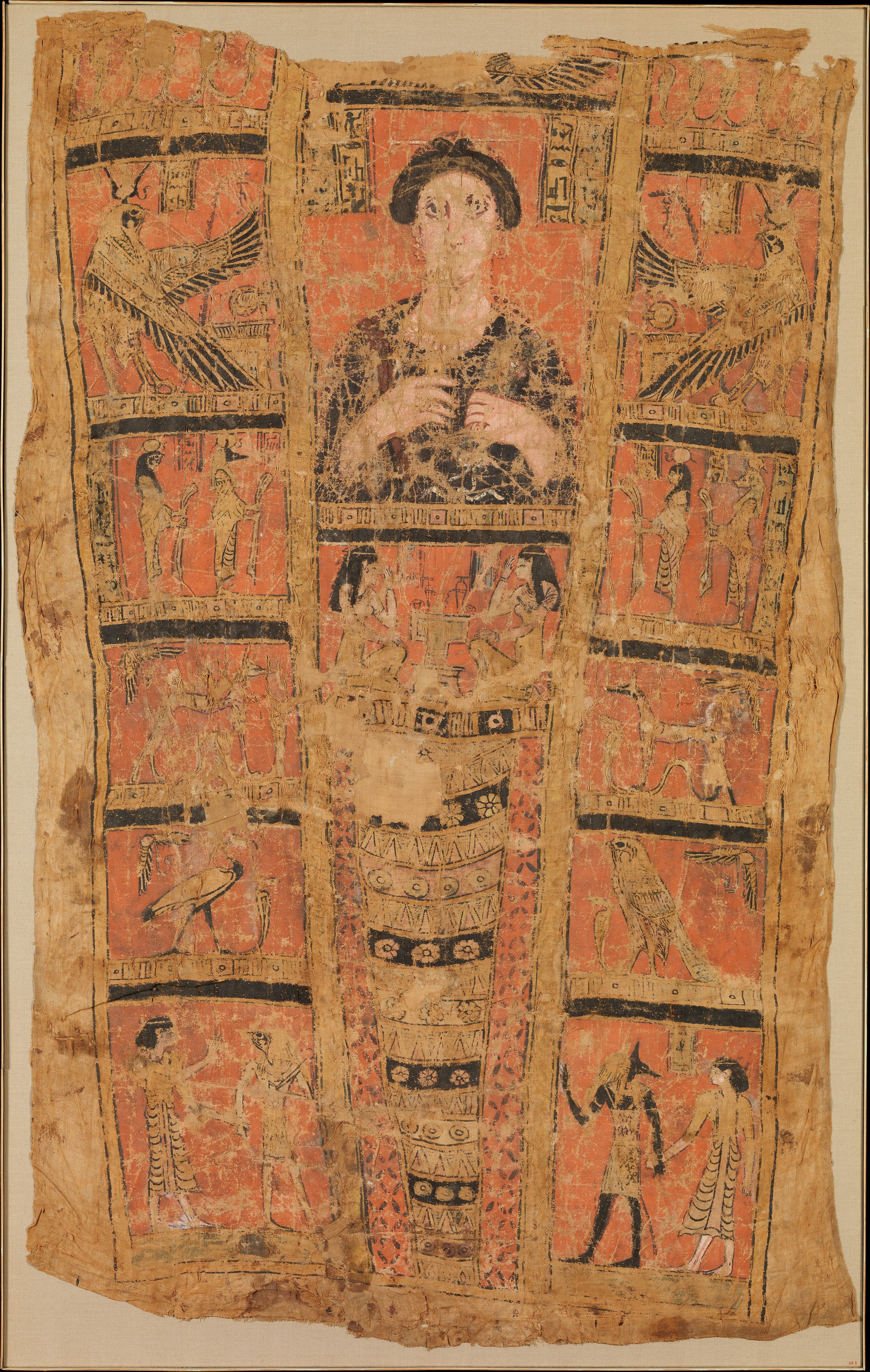This detailed photograph features a vintage tapestry with a yellowed, beige background, adorned with intricate hand-painted illustrations and hieroglyphics. The tapestry, which appears old and faded in areas, showcases various Egyptian gods, pharaohs, and mythical creatures, arranged in a rectangular grid pattern with distinct bordered panels. Each panel, bordered with black and gold lines and often featuring faded orange backgrounds, contains unique illustrations. At the top left, a half-bird, half-man with a crest on its head is depicted. Proceeding across the top, there are panels with gold eagles, each with wings outstretched and facing opposite directions. 

The middle sections include detailed paintings of pharaohs and gods, with some scenes showing a person in a long golden dress with black hair, standing with another figure, both holding a staff. In another panel, a creature resembling a horse with an elongated neck appears, drawn in gold and black. The central panel, notably, depicts a woman in an old-style Japanese kimono, emphasizing the multicultural influences within the tapestry's designs. 

Other panels feature various bird-like figures etched in gold and black ink, and mythical animals standing on human-like legs. Some of these illustrations are difficult to discern due to the tapestry’s age and wear, with parts of the fabric appearing folded, scratched, and torn. The overall piece is framed with a rough, tan border, giving it a rustic and antique appearance.